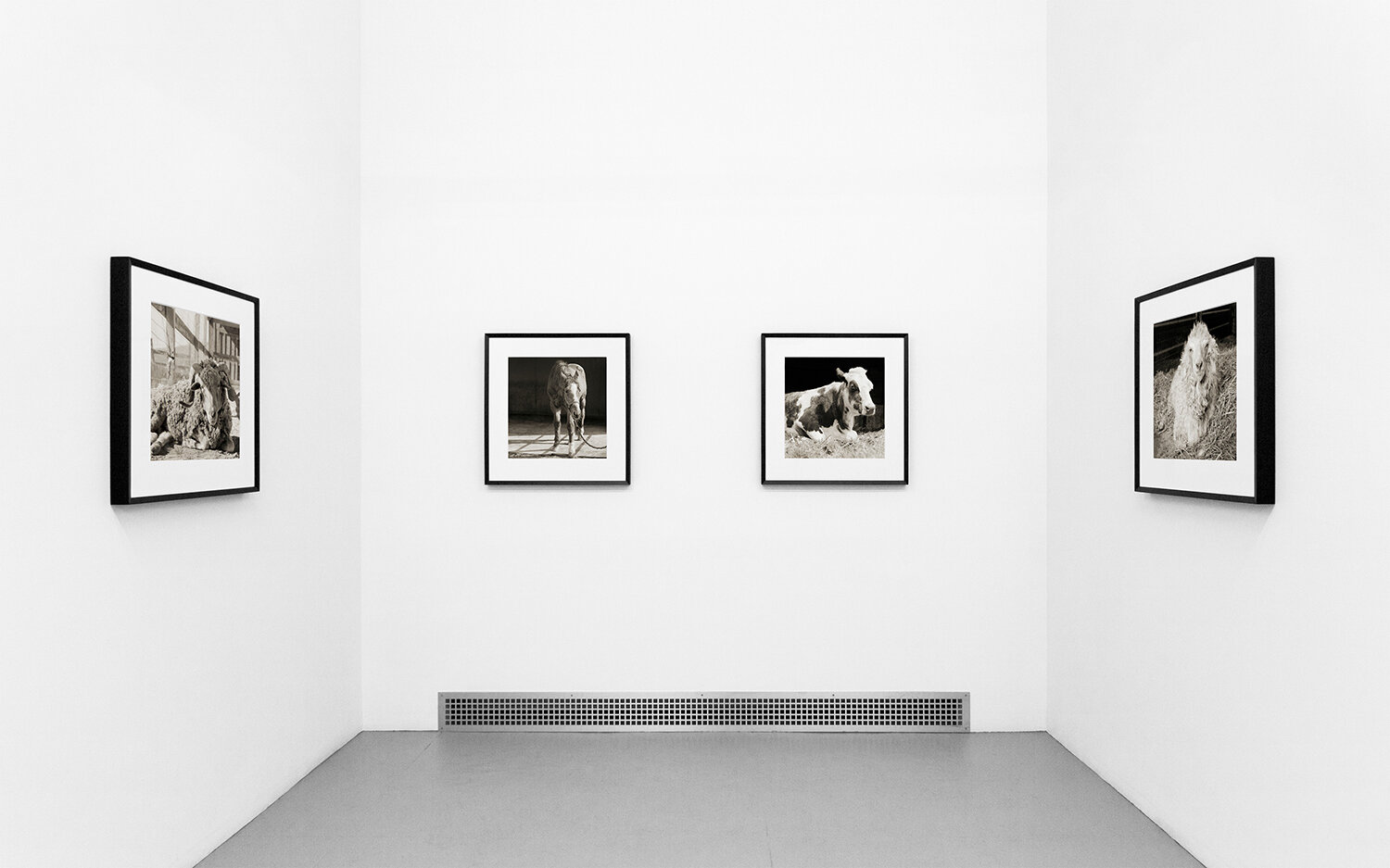This image showcases a minimalist room within a museum, featuring three pristine white walls and a gray floor. The walls are adorned with four black-and-white photographs of farm animals, each perfectly aligned at eye level. On the left wall hangs an image of a giant ram or goat, potentially resting with a bridge or enclosure bar in the background. The back wall features two images: the left one depicts a donkey with a rope attached to its bridle, its head slightly lowered, and the right one shows a cow either resting or behind a fence covered in growth. The right wall presents a smaller picture, likely of a sheep, ram, dog, or lamb. All photographs are encased in black frames with white borders, contributing to the room’s clean and sleek aesthetic. An air ventilation grill runs along the bottom of the back wall, enhancing the room's functional yet minimalistic design. There are no texts or additional furnishings, creating an exhibit that focuses entirely on the visual appeal of the animal photography.